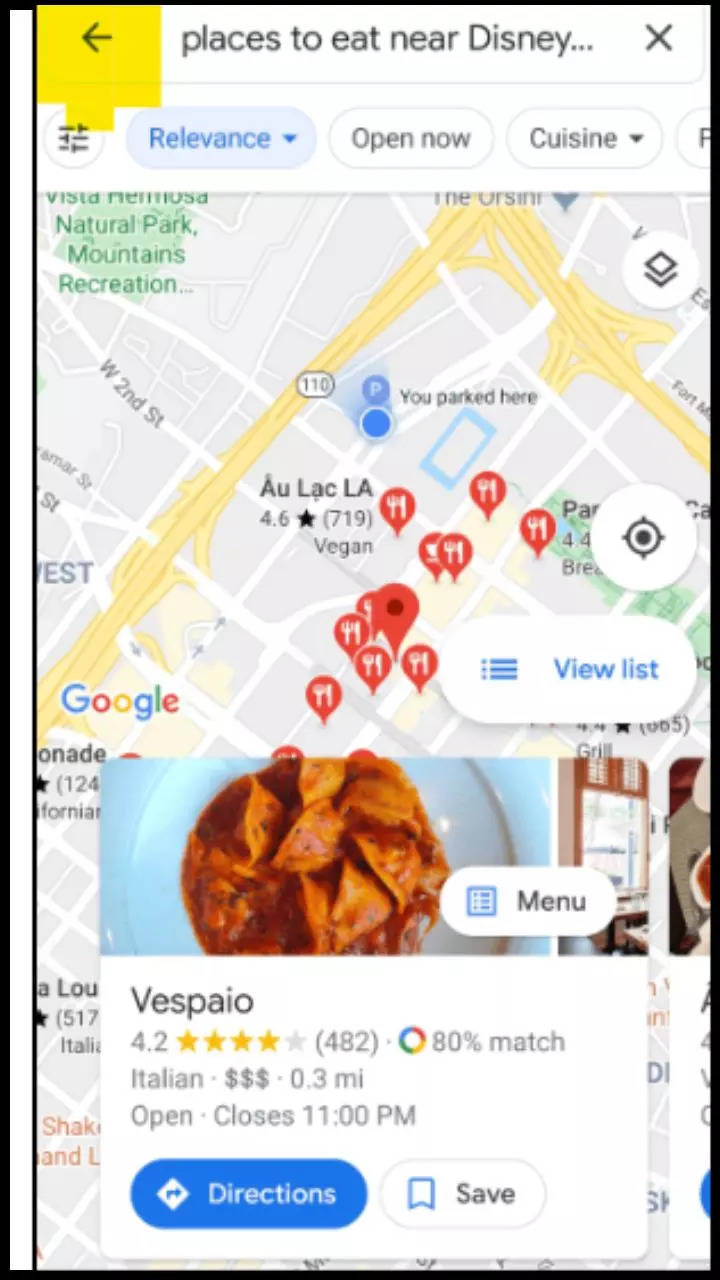This image is a detailed screenshot from someone's cell phone displaying a map search for dining options near Disney. 

- At the top left corner, there is a yellow box with a left-pointing arrow, likely a back button, next to a search bar containing the query "places to eat near Disney..." which is followed by an 'X' for clearing the search.
- Below the search bar, from left to right, there is a small circular icon with three horizontal lines, a blue button labeled "Relevance" indicating it is selected, a white button labeled "Open now," and another button marked "Cuisine."
- The main map section shows a highlighted area called Vista Hermosa Natural Park - Mountains Recreation on the left. A blue dot in the center of the map indicates "You parked here."
- Below the map, it says "All A-U-L-A-C-L-A" and a series of red markers with a white fork and knife icon, indicating the locations of various restaurants.
- There's a button labeled "View list" on the map.
- At the bottom, a specific restaurant entry for "Vespaio" is selected, featuring an image of a plate that appears to have raviolis. 
    - The listing shows a rating of 4.2 stars out of 5, with 482 reviews in parentheses and an 80% match to the search.
    - Its details are: Italian cuisine, indicated by three dollar signs to show the price range, located 0.3 miles away, currently open and closing at 11 p.m. 
    - Two buttons are available: a blue one labeled "Directions" and a white one labeled "Save."